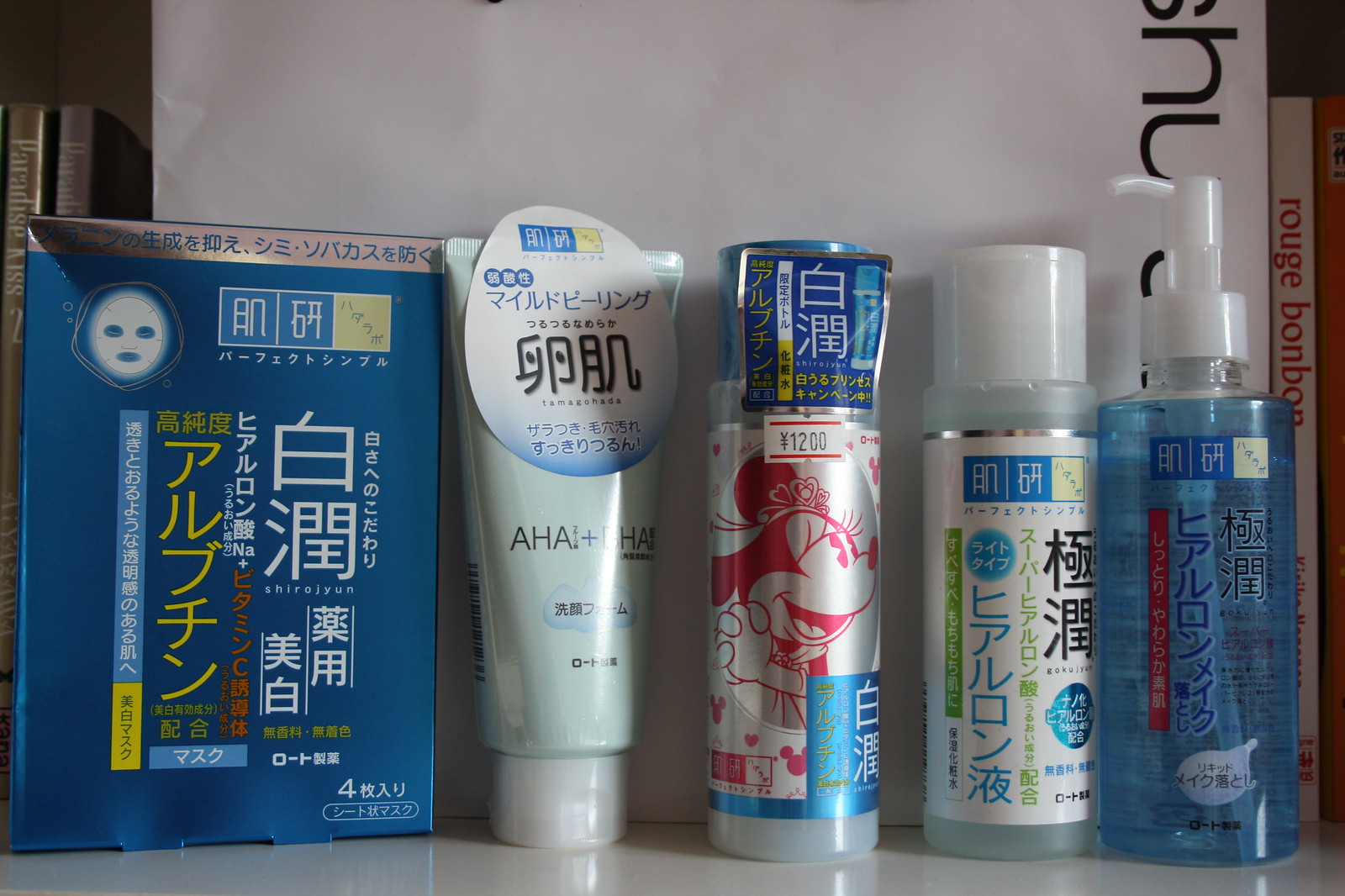A photograph captures an assortment of beauty products, predominantly in what appears to be Japanese packaging. The backdrop features a bookshelf with several items, one of which is a clearly readable book titled "Rouge Bonbon," while the titles of the remaining books are obscured. 

The first product on the left is a blue box, likely containing face masks as suggested by the small illustration on its front. Next to it is a bottle labeled with "AHA + BHA," indicating it might be a facial cleanser or exfoliant. The center bottle, priced at 1200 yen, is adorned with a whimsical design featuring Minnie Mouse surrounded by pink hearts and multiple smaller Mickey Mouse motifs, though its specific purpose remains unclear. 

The two rightmost bottles offer no hints about their contents, with one housed in a solid plastic container and the other in a clear bottle, revealing a blue liquid inside.